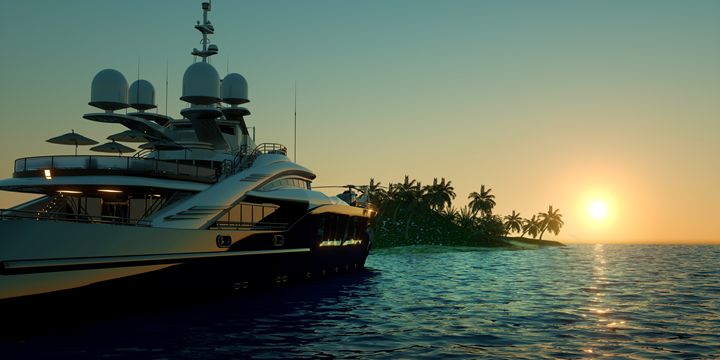This horizontal color photograph captures a serene sunset scene featuring a large yacht approaching an island. The yacht is prominently positioned on the left side of the image, facing the island with no visible people on board. It boasts four radar domes and several antennae on its top deck, along with two umbrellas suggesting an area for leisure. The yacht's hull appears to have a whitish-silver color on top and a darker shade, possibly black, on the bottom, with lights visible on the lower deck at the front.

The water, seen on the lower right, is calm and reflects the setting sun, which is almost touching the horizon. The sky above transitions from a dark blue at the top to rich shades of orange and yellow near the horizon. The sun casts a beautiful reflection on the water, enhancing the tranquility of the scene.

In the background, just to the left of the setting sun, lies the island adorned with several silhouetted palm trees, adding to the tropical ambiance. The overall composition merges the vibrant colors of the sunset with the tranquil blues of the ocean and sky, creating a picturesque and peaceful moment.